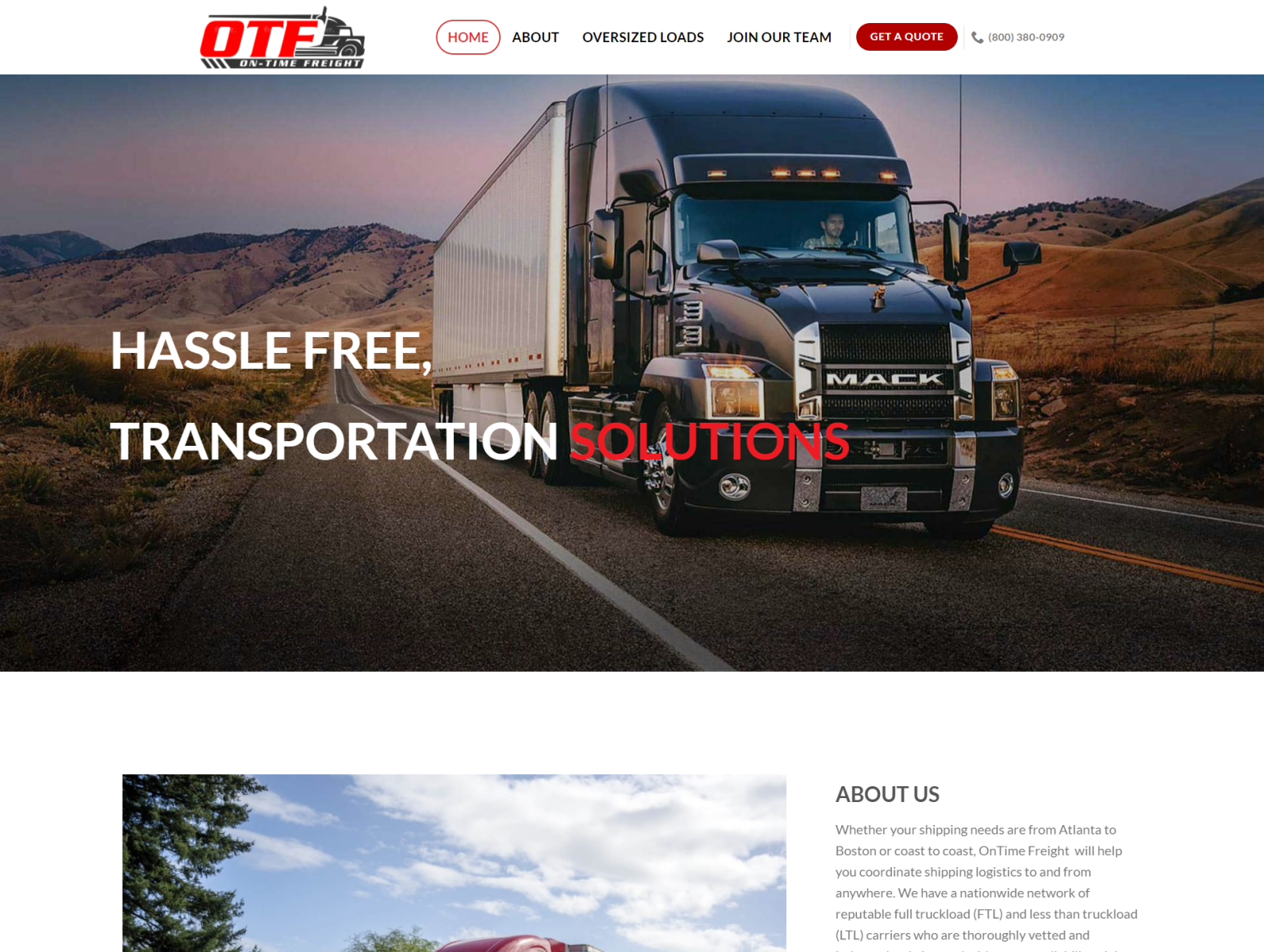The image showcases the homepage of a photographer's website featuring the logistics company, On Time Freight (OTF). In the upper left-hand corner, the company logo—red letters "OTF" encapsulated within the shape of a tractor-trailer—prominently displays the brand identity. The navigation menu at the top includes options like Home, About, Oversize Loads, Join Our Team, Get a Quote, and a phone number with a telephone icon beside it. 

The Home button is highlighted within a white circle outlined in red, featuring red text, while the "Get a Quote" button stands out in a solid red bubble with white text. Below the menu, a large horizontal banner image spans the width of the homepage. This image features a robust Mack semi-truck traveling through a desolate, hilly, desert landscape, evocative of the Southwestern United States. 

Superimposed on the image, white text reads "Hassle-Free Transportation Solutions," with the word "Solutions" emphasized in red. Below this, an "About Us" section states, "Whether your shipping needs are from Atlanta to Boston or coast to coast, On Time Freight will help you coordinate shipping logistics to and from anywhere. We have a nationwide network of reputable, full truckload (FTL) and less than truckload (LTL) carriers who are thoroughly vetted."